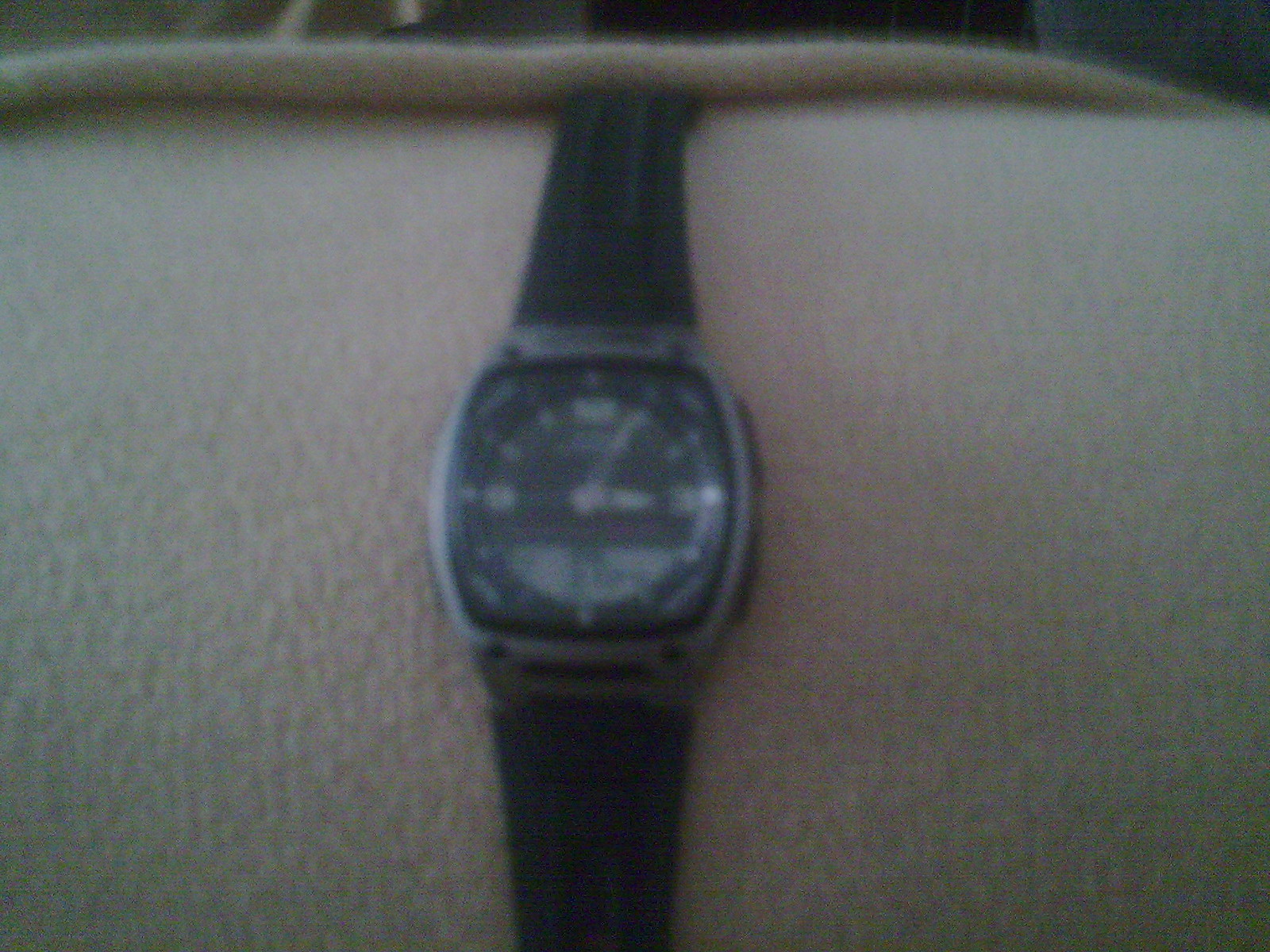This image features a wristwatch elegantly displayed on a beige fabric. The watch has a unique, square-like face with subtly bulged sides, creating a distinctive aesthetic. The watch face is black, adorned with minimalist white numerals at the 12, 3, 6, and 9 o'clock positions, while the other hour markers are represented by simple white ticks. The hands of the watch are also black, adding a refined contrast against the dark background. Completing the sleek design, the watch strap is black, contributing to the overall sophisticated appearance of the timepiece.